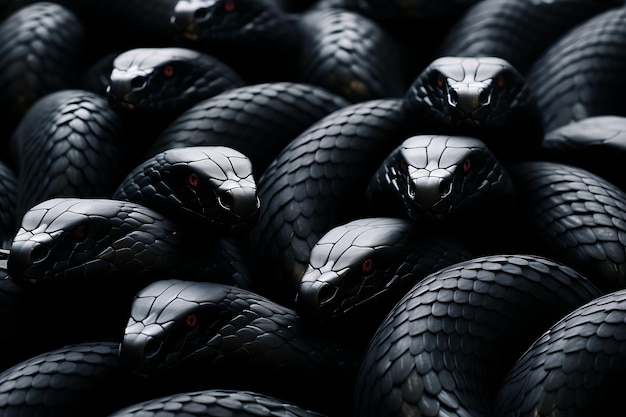In the image, a meticulous 3D artist's render showcases an intricate tangle of black snakes, each with scales resembling sharp, reflective ovals that cover their entire bodies, giving off a shiny, charcoal-like appearance. The snakes' eyes are a dull red with black pupils, exuding a menacing vibe akin to vipers, further heightened by their pronounced nostril pits. The scene is dominated by this knot of snakes, creating an almost surreal and artificial effect, with eight snake heads prominently emerging from the intertwined bodies. Seven of these heads are oriented towards the left at the bottom, while one centrally located head slightly to the left is facing right. An additional snake head is barely visible peeking out from the background on the left. The overall composition signifies a dense and visually compelling mass of serpentine forms, reminiscent of something out of an Indiana Jones adventure, emphasizing the meticulously crafted and uncanny nature of the depiction.